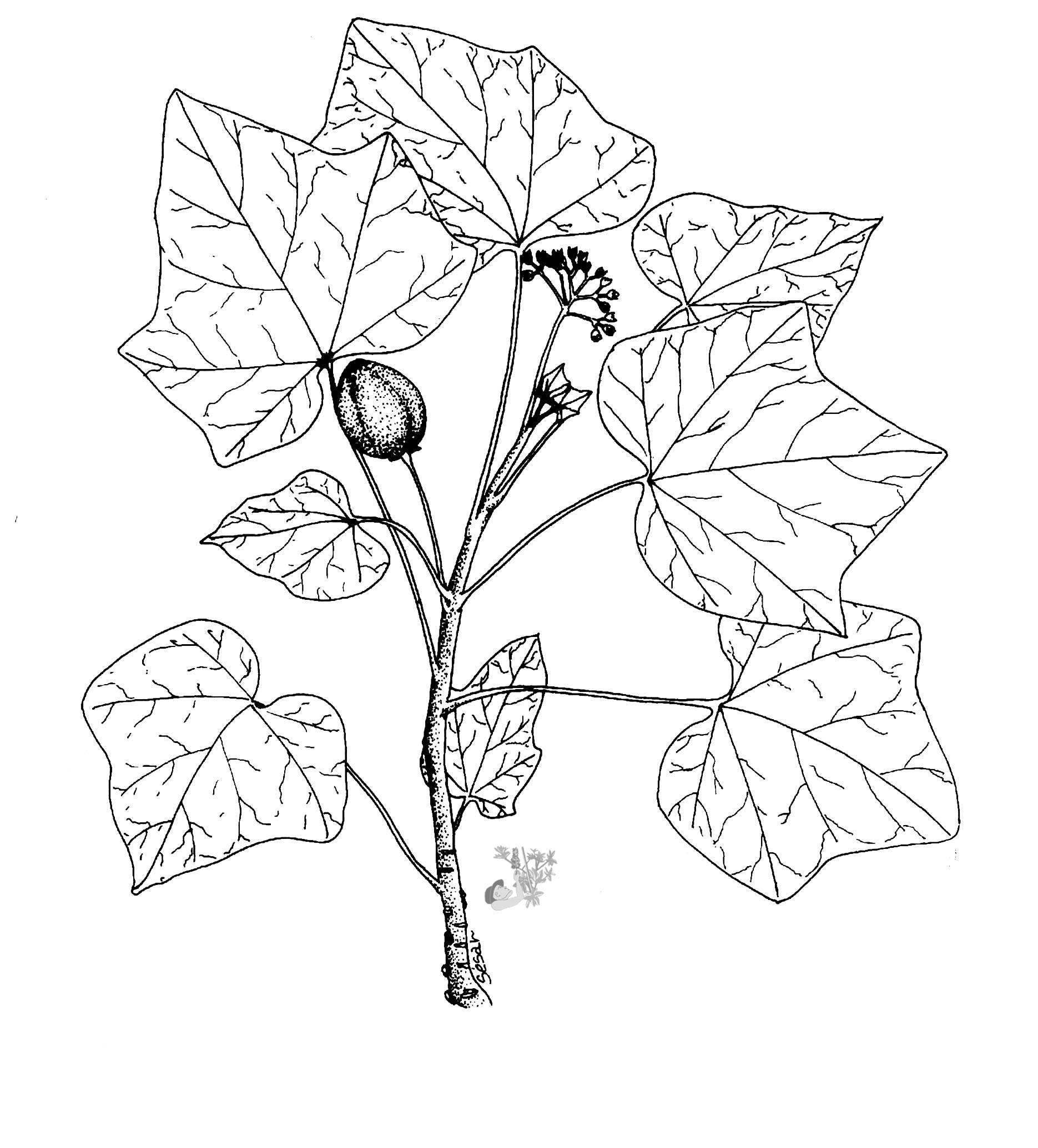This finely detailed pencil drawing depicts a plant with a central stem rising from the base, adorned with an array of leaves varying in size. The leaves, reminiscent of either ivy or oak, exhibit a web-like structure with three to five points and intricate vein patterns radiating from the center. The stem branches out midway into a bulbous structure and culminates in a cluster of flower pods at the top. Aside from the plant, there's a faint, separate illustration of a person wearing a hat, seemingly holding a smaller version of the plant. The entire artwork is rendered in black and white, with the signature "Caesar" inscribed at the bottom.